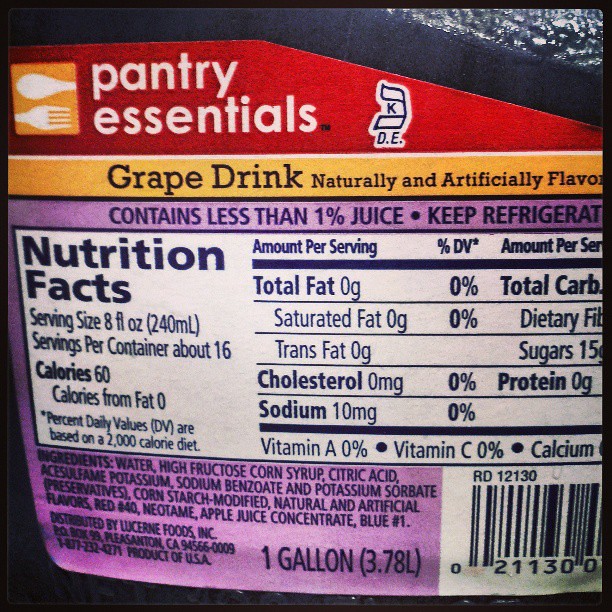This image showcases a detailed label from a food product. At the top, the label features a red section with a minimalist illustration of the upper parts of a spoon and a fork, accompanied by the text "Pantry Essentials." Directly below this, there's an orange stripe highlighting the product type: "Grape Drink, Naturally and Artificially Flavored." Following this, a purple stripe provides additional product information: "Contains Less Than 1% Juice, Keep Refrigerated." The nutrition facts section is prominently displayed beneath these descriptions. It specifies a serving size of 8 fluid ounces (240 ml), with approximately 16 servings per container. Each serving contains 60 calories, with no calories from fat (*% Daily Values (DV)).